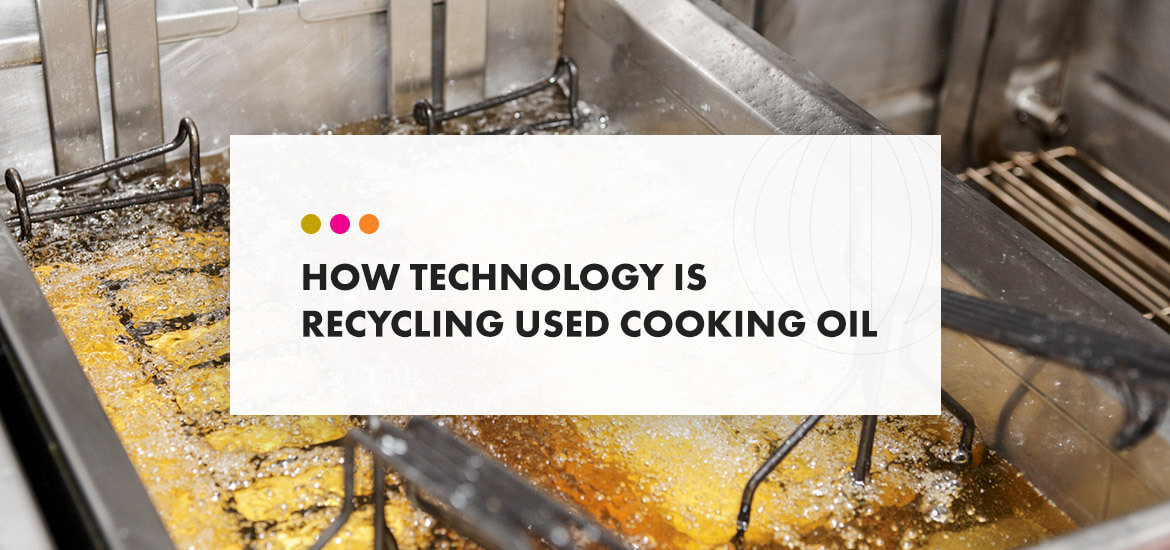The image prominently features an industrial deep-fat fryer with two metal baskets submerges in oil. The fryer, constructed from shiny metallic material, has a silver hue and involves a noticeable empty oil section beside the filled one. The scene appears somewhat messy, reminiscent of oil-laden trays inside an oven. Superimposed centrally on this photograph is a white, semi-opaque text box, occupying approximately one-third of the image. Bold black capital letters within the box read, "HOW TECHNOLOGY IS RECYCLING USED COOKING OIL." Just above the text, three horizontally-aligned circles add a splash of color: one beige, one pink, and one orange. This composition effectively emphasizes the concept of recycling used cooking oil through technology.